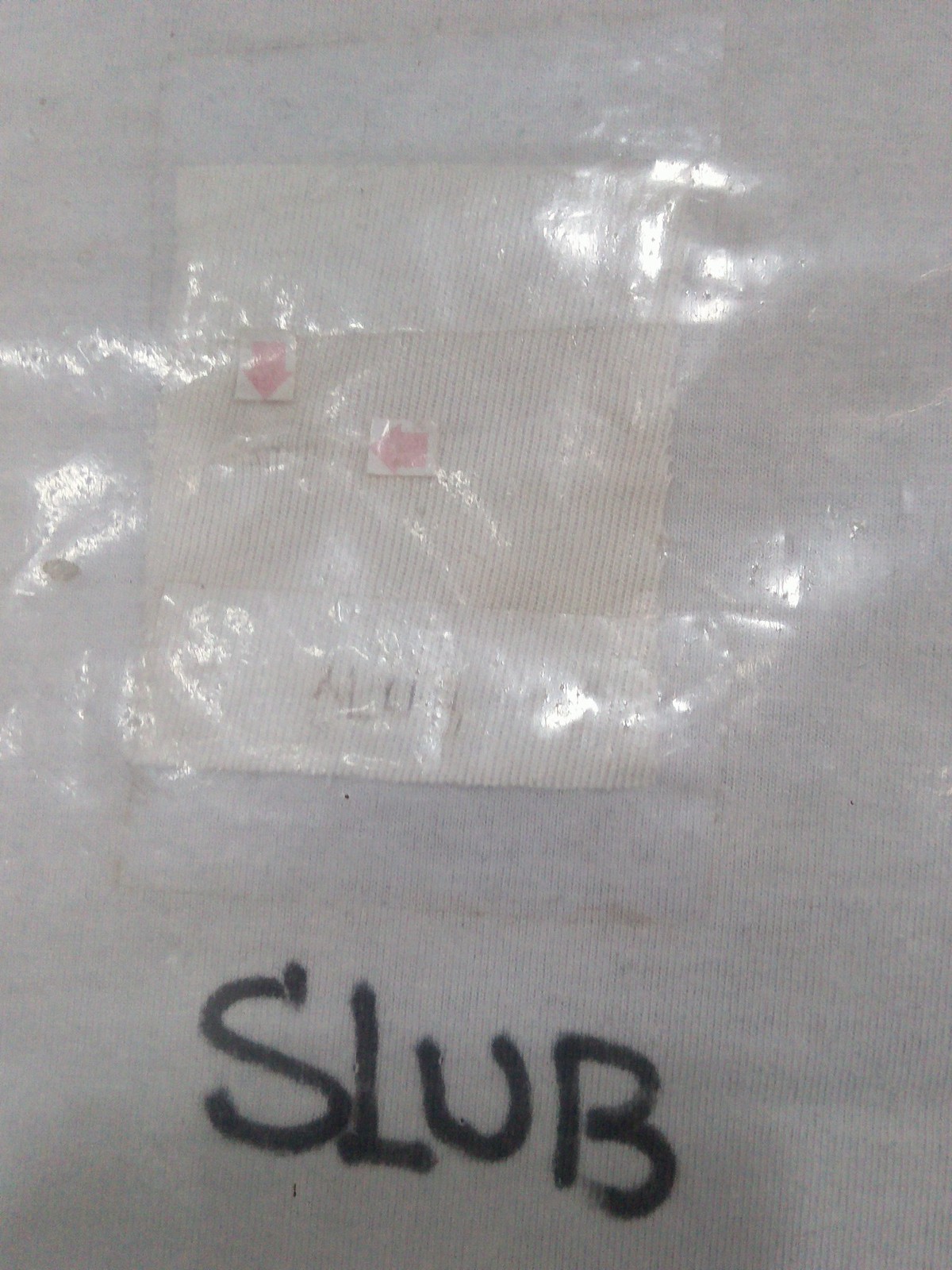This is an intricate graffiti drawing on a wall, featuring the word "SLUB" prominently in bold, black capital letters. Above the graffiti, there appears to be a large piece of clear tape affixed to the wall. Directly below the word "SLUB" is an off-white bag, adorned with a couple of arrow tabs indicating points of access. The top part of this bag shows rolled-down edges or significant creases in the plastic. Additionally, there are some pencil-drawn initials or letters, "A-L-U," on the bag, further adding to the complexity of the scene.